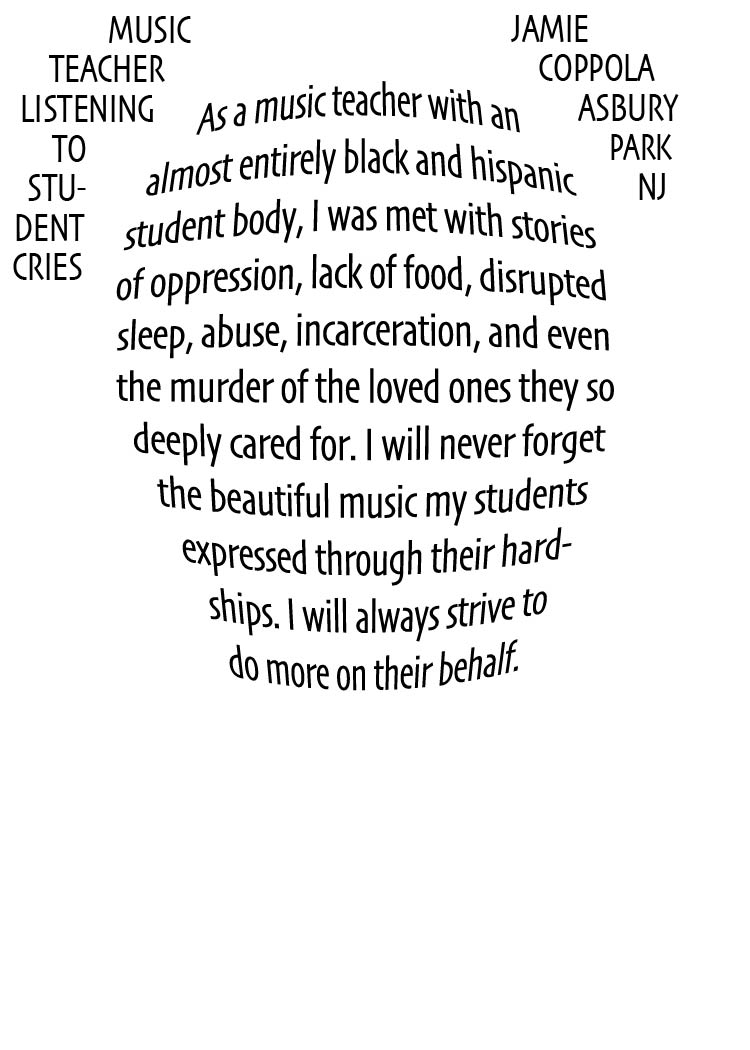This digitally synthesized image features a plain white background with black, capitalized text. At the center is a somewhat circular shape, tapering at both the top and bottom, and constructed entirely from words. These words form a poignant narrative: "As a music teacher with an almost entirely Black and Hispanic student body, I was met with stories of oppression, lack of food, disrupted sleep, abuse, incarceration, and even the murder of loved ones they so deeply cared for. I will never forget the beautiful music my students expressed through their hardships. I will always strive to do more on their behalf." This central text appears slightly rotated on the sides, giving it a three-dimensional effect. Curving around the top left of the central shape, the text reads "Music Teacher Listening to Student Cries," creating an artistic representation that evokes the image of ears and a face. On the right side, another inscription reads, "Jamie Coppola, Asbury Park, New Jersey," attributing the work to the artist.